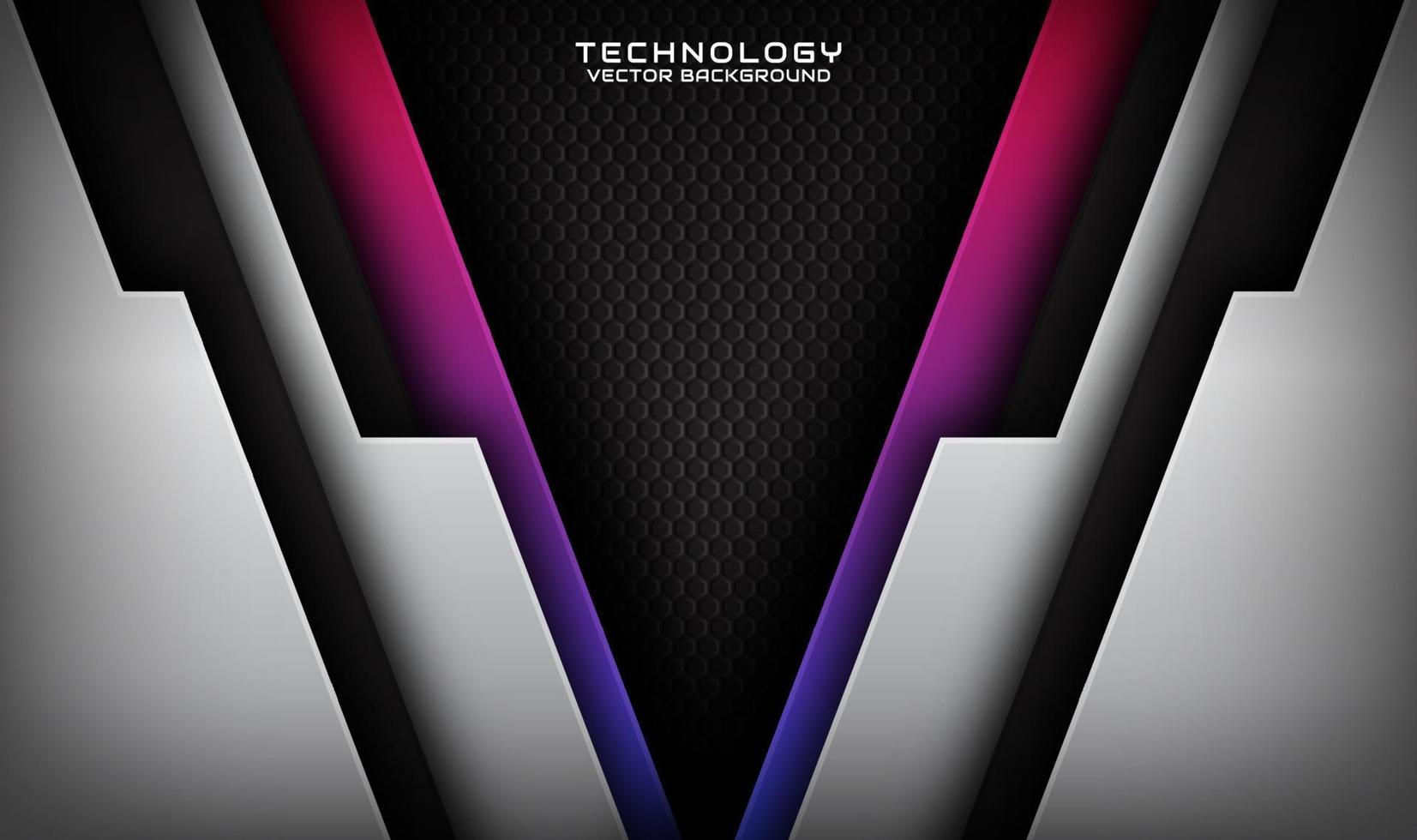The image features a striking vector background with a central white text that reads "Technology Vector Background." The text is set against a black V-shaped background filled with a hexagonal grid pattern. Flanking this central element are inclined rectangular bars forming a larger V-shape, with a smooth gradient transitioning from pink at the top to purple at the bottom. Beyond these, there are additional panels shaped to create a three-dimensional effect; these panels are primarily silver or gray, intersected with black. The overall image has an arresting color scheme of gray, black, fuchsia, purple, and white, combining to provide a dynamic and technologically sophisticated appearance.